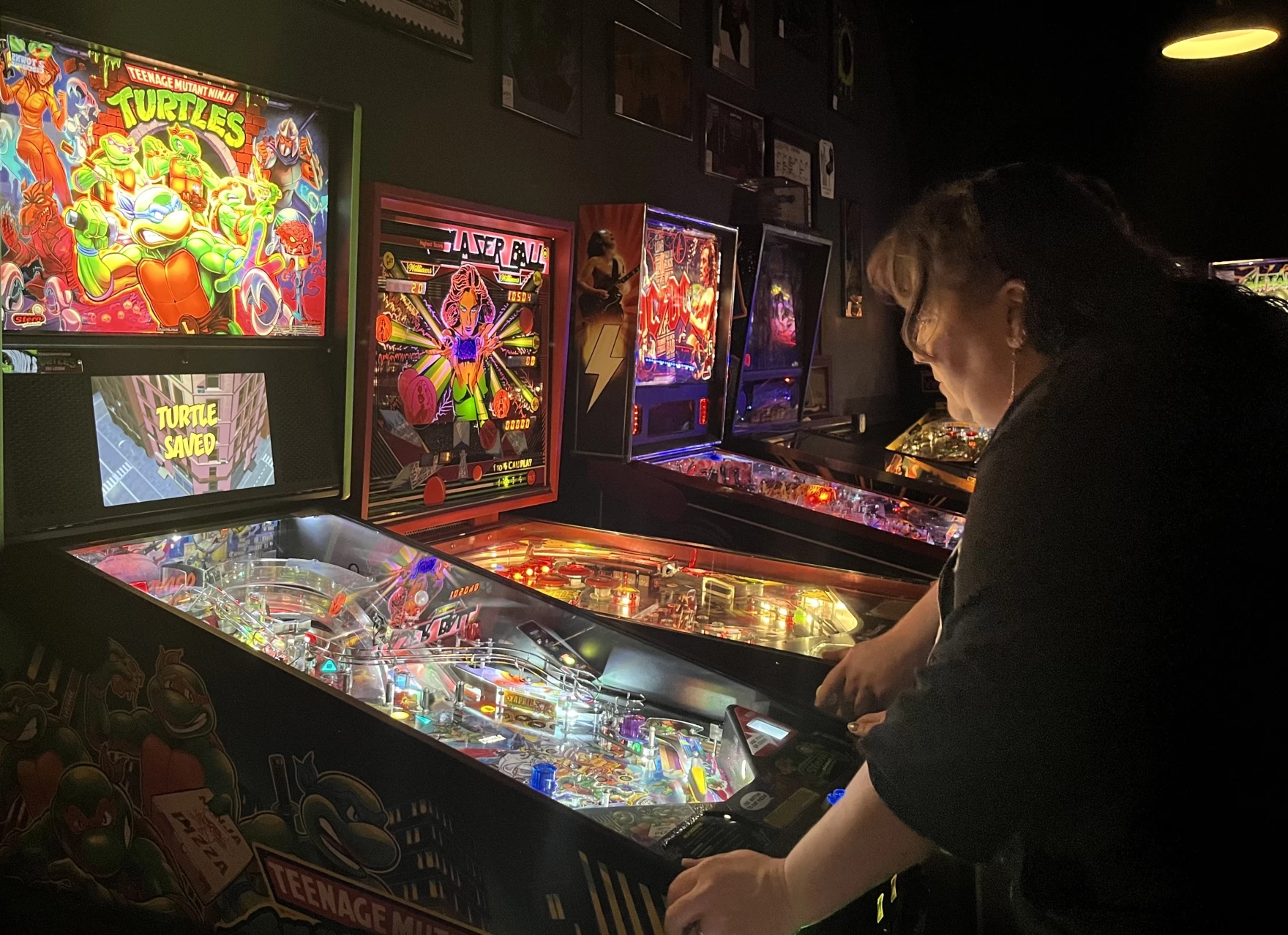In this dimly lit arcade, an individual, who appears to be overweight with brown hair and an earring on the left ear, is intently playing a Teenage Mutant Ninja Turtles pinball machine. This retro machine prominently displays an image of the iconic 1990s cartoon characters—green, human-like turtles wielding weapons, alongside April, the reporter, in her signature orange outfit. The machine's screen flashes "Turtle Saved." Flanking the Ninja Turtles pinball are other vintage machines, including "Laser Ball" and an AC/DC-themed one. The arcade's walls are a mix of green and black, adorned with paintings and pictures, and illuminated by neon lights in vibrant hues of blue and red.